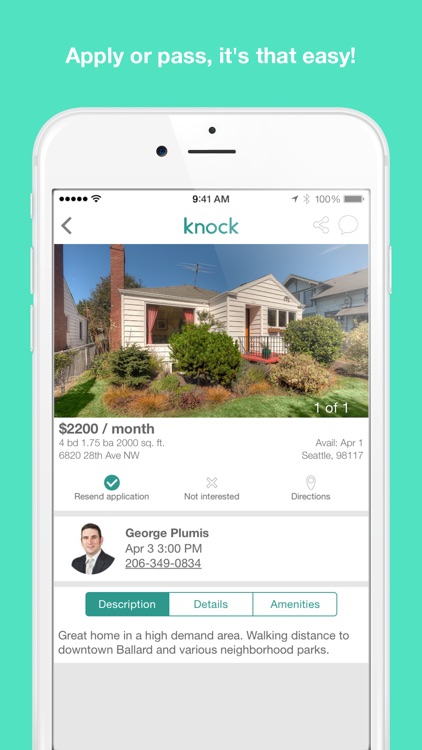This ad is a vertical, rectangular display ad likely sourced from a website. The background is aquamarine green, and the heading at the top reads in white text: "Apply or Pass. It's that easy." Directly beneath this, there's an image of a smartphone displaying a website named "KNOCK" in blue font against a white backdrop.

The smartphone's screen shows a photo of a light beige, single-story suburban house adorned with plentiful bushes and set in a well-maintained front yard. Below the house image, details of the property are listed: a rental rate of $2,200 per month for a four-bedroom, 1.75-bathroom home spanning 2,000 square feet. The address is given as 6820 28th Avenue Northwest.

Further down, there is a headshot of the real estate agent, George Plumas, a man in his 30s with dark brown hair, dressed in a white shirt, light-colored tie, and black suit. An April 3rd appointment time is noted at 3:30, accompanied by a contact phone number.

To round off the ad, a brief property description is provided at the bottom: "Great home in a high-demand area, walking distance to downtown Ballard and various neighborhood parks."